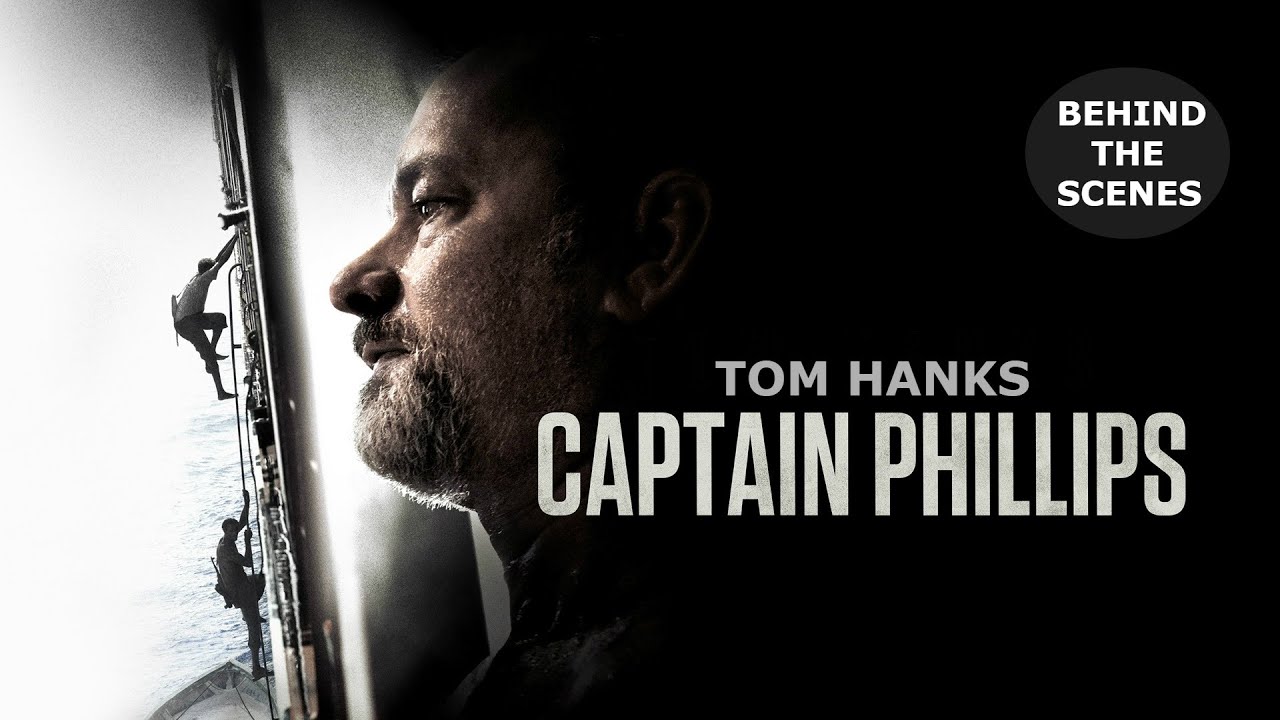This horizontally rectangular movie poster for "Captain Phillips" prominently features Tom Hanks. The right side of the image is dominated by a black background with white text in the upper right-hand corner reading "BEHIND THE SCENES". Below that, more centrally placed, are the names "Tom Hanks" in gray text and "Captain Phillips" in bold white text. The left side is brighter, showcasing a partial profile of Tom Hanks, who sports a gray beard and gazes off to the left. Adjacent to his face, the scene reveals two pirates climbing a ladder on the side of a ship, with the ocean and the ship's bow faintly visible in the background. The overall composition merges a sense of tension and focus, serving as an evocative promotional piece for the intense maritime thriller.